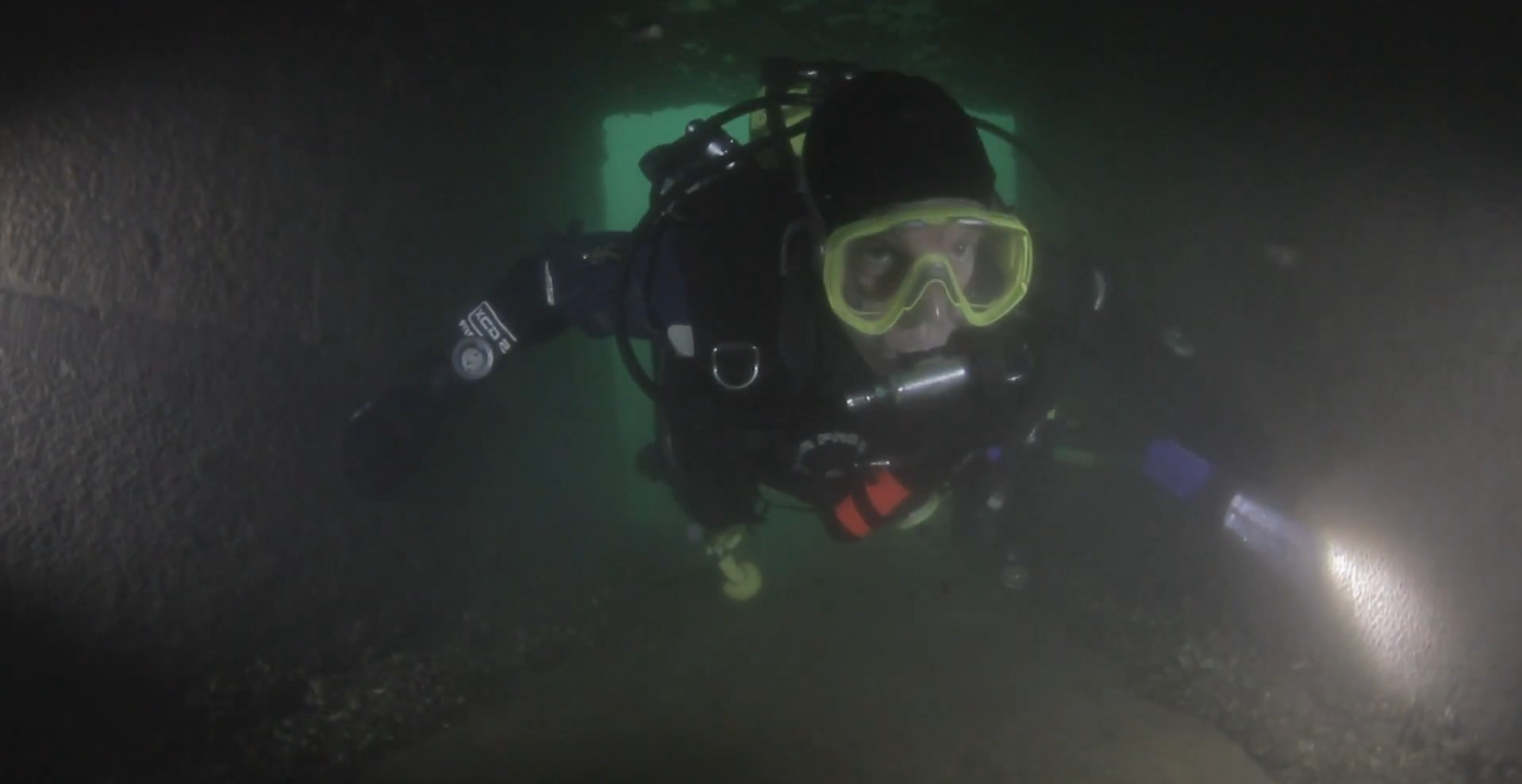This color photograph, taken underwater in a landscape orientation, captures a white male scuba diver in a murky, dark green environment. The image depicts the diver in mid-swim, moving straight ahead and parallel to the seafloor. He is equipped with black scuba gear, including a wetsuit, and yellowish-green goggles. A dark blue tank is strapped to his back. The diver's left hand holds a flashlight, which illuminates the left wall of what appears to be a tunnel, cave, or possibly a sunken ship. His eyes are open and staring forward through the light reflective water, casting a light green hue in the background.